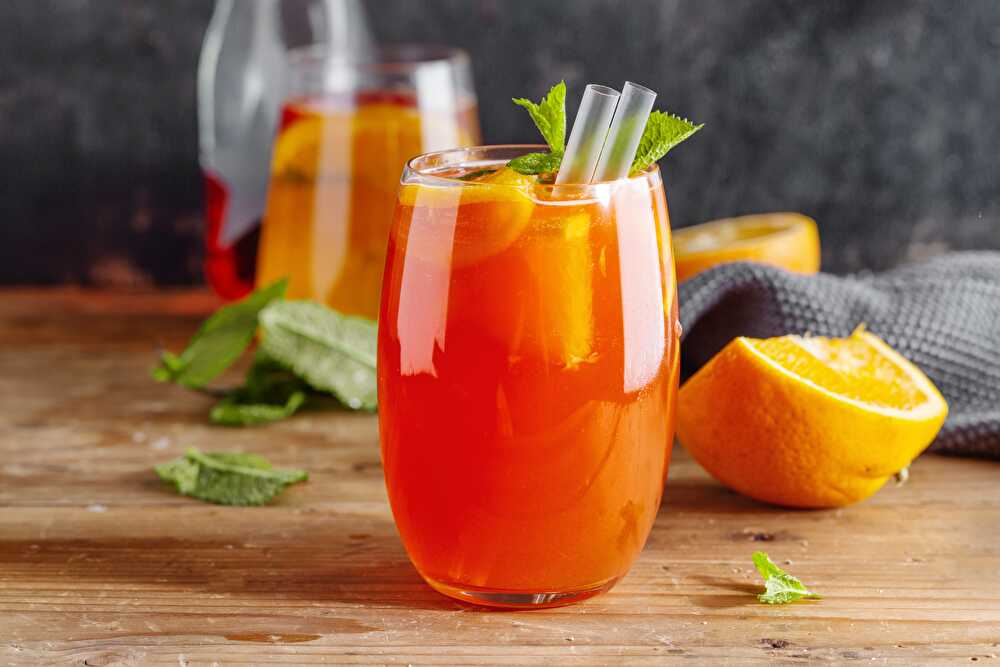This vibrant horizontal color photo prominently features a bright orange drink set in a clear, oval-shaped glass. The drink, filled to the brim, contains fresh orange slices and sprigs of mint, with two straws sticking out of the top. The glass is set on a light wooden table, which also hosts scattered torn mint leaves and two cut orange halves to the right of the main glass. A dark gray towel partially covers the table near the oranges. In the background, which is artfully blurred, you can discern a second similar glass of the same orange drink without straws or mint, flanked further back by a pitcher adorned with a star, presumably for refilling the drinks. The entire setup is beautifully contrasted against a speckled gray and black background, adding to the overall rustic yet refreshing feel of the image.